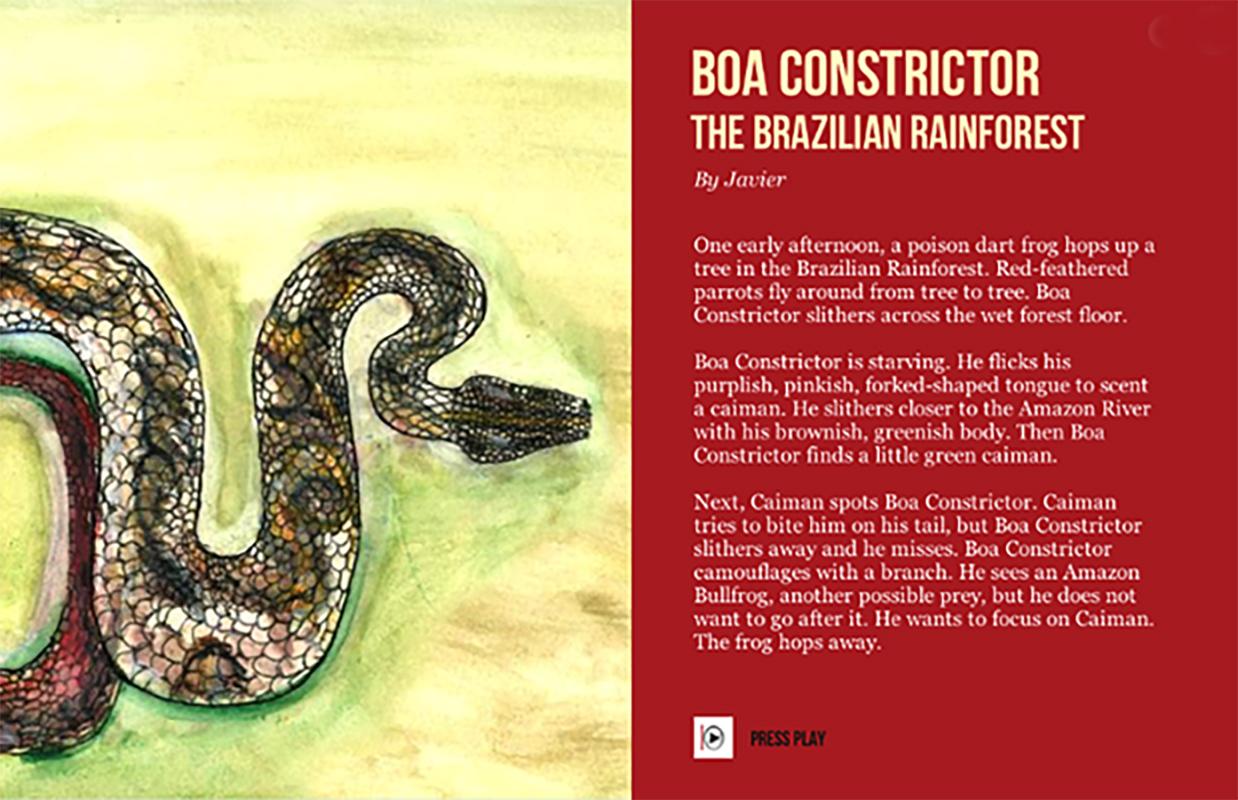The image is an informational poster divided into two sections. On the left side, there is a colored drawing of a boa constrictor. The snake starts from the top middle of the left section, curling its way down and to the right, then down again, moving back up, to the left, and finally, right where its head is located in the middle right of the section. This large snake is light-colored with dark markings and has an arrowhead-shaped head. Additionally, there is a smaller reddish-colored snake beneath the larger one's starting point, entering from the left edge, moving slightly right, down, and exiting off the bottom of the left edge. The background of this section is a mix of beige and green hues.

On the right side of the poster, set against a red background, "Boa Constrictor" is written in large beige letters at the top. Below that, in slightly smaller print, is "The Brazilian Rainforest" and then in even smaller print, "by Javier". Following this, there are three paragraphs of detailed text, narrating a story: one mentions a poison dart frog hopping up a tree, another red feathered parrots flying from tree to tree, and the boa slithering across the forest floor. At the bottom left corner of this section, there is a white square with a symbol in it, next to the words "press play" in black writing.